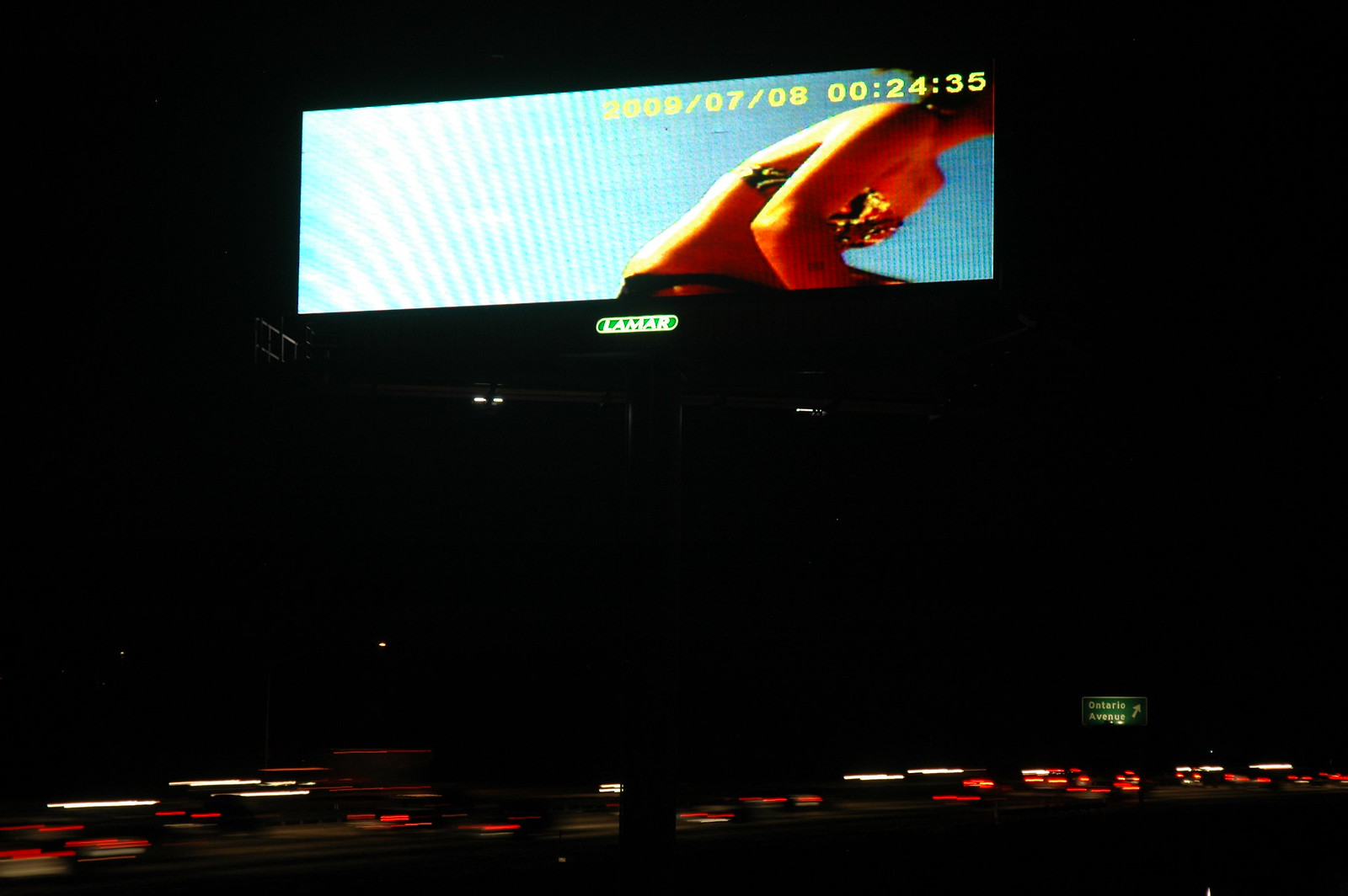This photograph captures a dark, dimly lit scene dominated by shadows and obscurity. The primary feature within the image is a digital screen situated slightly off-center towards the left and horizontally wider than it is tall. The screen exhibits a blue background and partially displays the torso of an individual wearing a bikini top or bra along with shorts, although the person's head is cut off at the top edge of the screen.

Above the torso, the screen features yellow text reading "2009/07/08 00:24:35," likely indicating the date and time the image or video still was captured. A small green circle below this text contains the word "Lamar," possibly denoting the brand or a label, although its exact significance remains uncertain due to the overall blur and darkness that envelopes the rest of the photo.

Additionally, at the bottom of the photograph, there are faint red and white lights providing subtle illumination. The majority of the image, however, remains enveloped in shadows, making it difficult to discern further details or context.